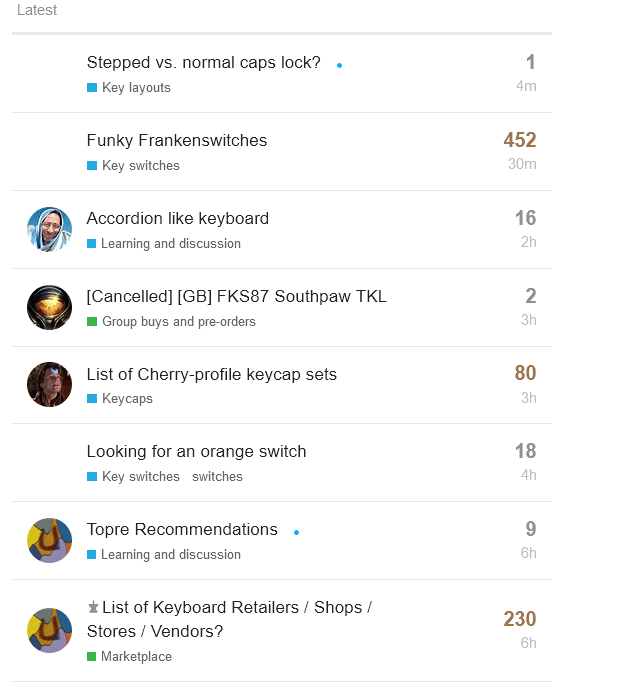The image appears to be a forum display with a list of recent discussion topics along with timestamps and participant counts. Here is a detailed descriptive caption of the image:

---

The image depicts a forum's "Latest" discussions section, organized in chronological order by the most recent activity. Each entry includes a topic title, category, and participation metrics. Here are the details:

1. **Topic:** "Stepped vs Normal Caps Lock?"  
   - **Time:** 4 minutes ago  
   - **Category:** Key Layouts (represented by a blue square)  
   - **Participants:** 1
  
2. **Topic:** "Funky Franken Switches"  
   - **Time:** 30 minutes ago  
   - **Category:** Key Switches (represented by a blue square)  
   - **Participants:** 452

3. **Topic:** "Accordion Light Keyboard"  
   - **Time:** 2 hours ago  
   - **Category:** Earning Discussion (represented by a blue square)  
   - **Participants:** 16  
   - **Profile Picture:** A white man wearing glasses and a blue hoodie

4. **Topic:** "GBFKS87 Southpaw TKL"  
   - **Time:** 3 hours ago  
   - **Category:** Group Buys for Pre-orders (represented by a green square)  
   - **Participants:** 2  
   - **Profile Picture:** A gaming character, possibly an astronaut

5. **Topic:** "List of Cherry Profile Keycap Set"  
   - **Time:** 3 hours ago  
   - **Category:** Key Caps (represented by a blue square)  
   - **Participants:** 80
  
6. **Topic:** (Additional entries mentioned without complete details)  
   - **Times ranging from 4 to 236 hours ago** 

The forum covers varied topics such as key layouts, key switches, earnings discussions, group buys, pre-orders, key caps, and more, all pertaining to the keyboard community. The categories are visually distinguished by colored squares, with some posts featuring user profile pictures.

---

This caption provides a comprehensive description of the forum's latest discussion topics, including categories, participation details, and notable features of certain posts.